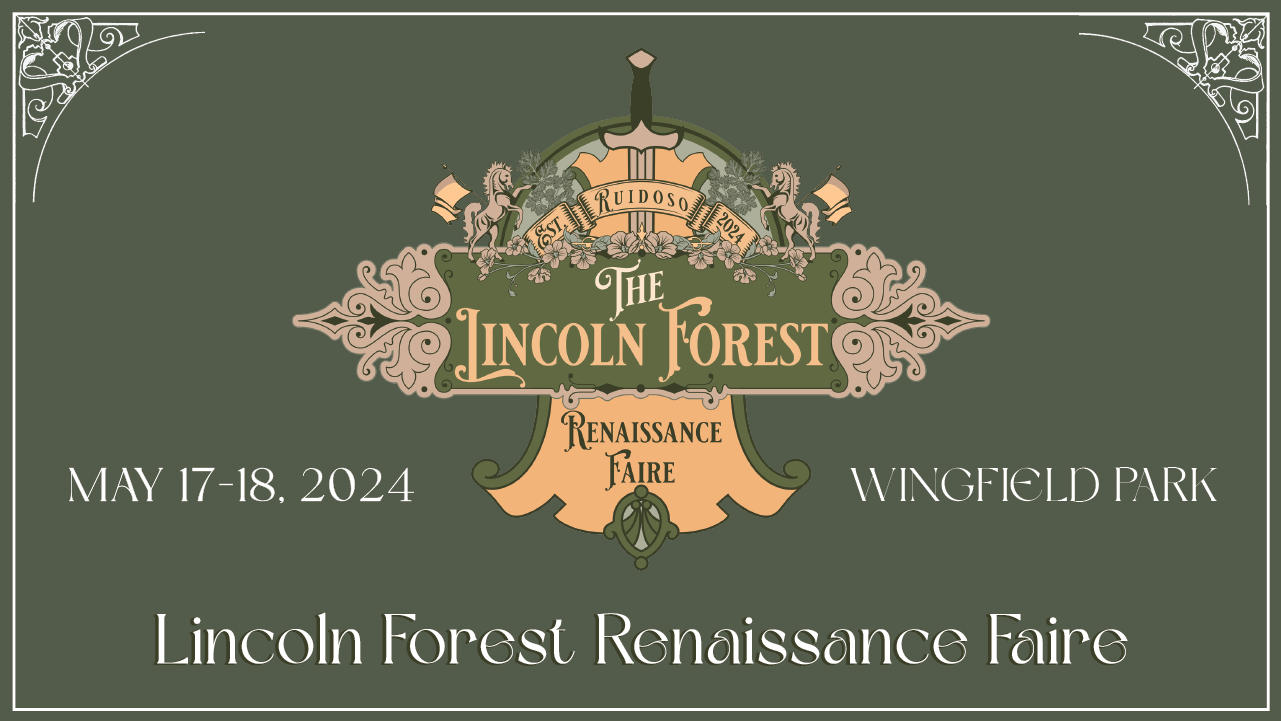This image is a landscape-format flyer or sign for a Renaissance fair, adorned with ornate, vintage-inspired elements. The background is a rich, dark green, bordered by a white line framing the entire rectangle. In the top left and right corners, intricate scrollwork details, featuring half and quarter circles, add an elegant touch.

Dominating the center is an old-world design that catches the eye immediately. At the top of this centerpiece is a semicircle flanked by two majestic unicorns. A ribbon with a motto unfurls gracefully, surmounted by a sword hilt with the blade extending downwards through the central motif. The inscription "The Lincoln Forest" is emblazoned in the middle, set against a slightly different green background and rendered in white and goldish-yellow lettering. The borders of this central rectangle feature scrolled points extending left and right, enhancing the flyer’s decorative appeal.

Below this central theme, a flared ribbon detail stands out, announcing "Renaissance Fair" in green text against a goldish-yellow backdrop. In white, block capital letters to the left of the ribbon, the dates "May 17 to 18, 2024" are clearly displayed. To the right, the location "Wingfield Park" is specified. At the bottom of the flyer, the full title "Lincoln Forest Renaissance Fair" is prominently featured, completing the design with a touch of medieval charm.